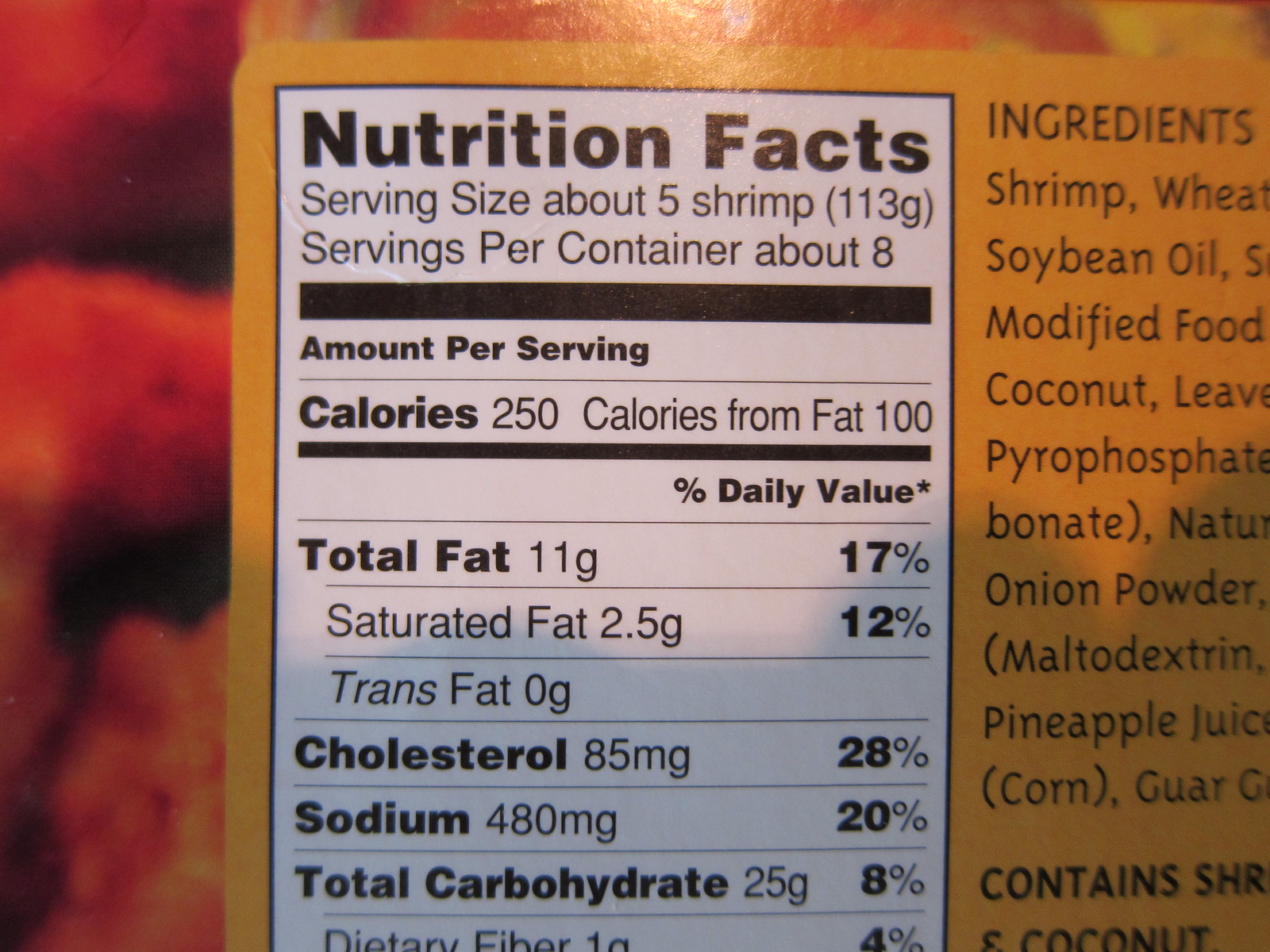This image depicts a nutritional facts label for a food product that contains shrimp and possibly coconut. The serving size is approximately 5 shrimp, with about 8 servings per container. Each serving provides 250 calories, with 100 calories derived from fat. The total fat content is 11 grams, including 2.5 grams of saturated fat, and there is no trans fat. The cholesterol content is unspecified. The product also contains sodium and total carbohydrates amounting to 25 grams. The label indicates that the food could be a jarred or bagged item, but suggests a jar due to its see-through nature. The product appears to be something with shrimp and might have a reddish component, possibly red beets or red peppers, but the exact nature of the red ingredient is unclear. Overall, the label suggests a dish involving shrimp and coconut, potentially coconut shrimp.